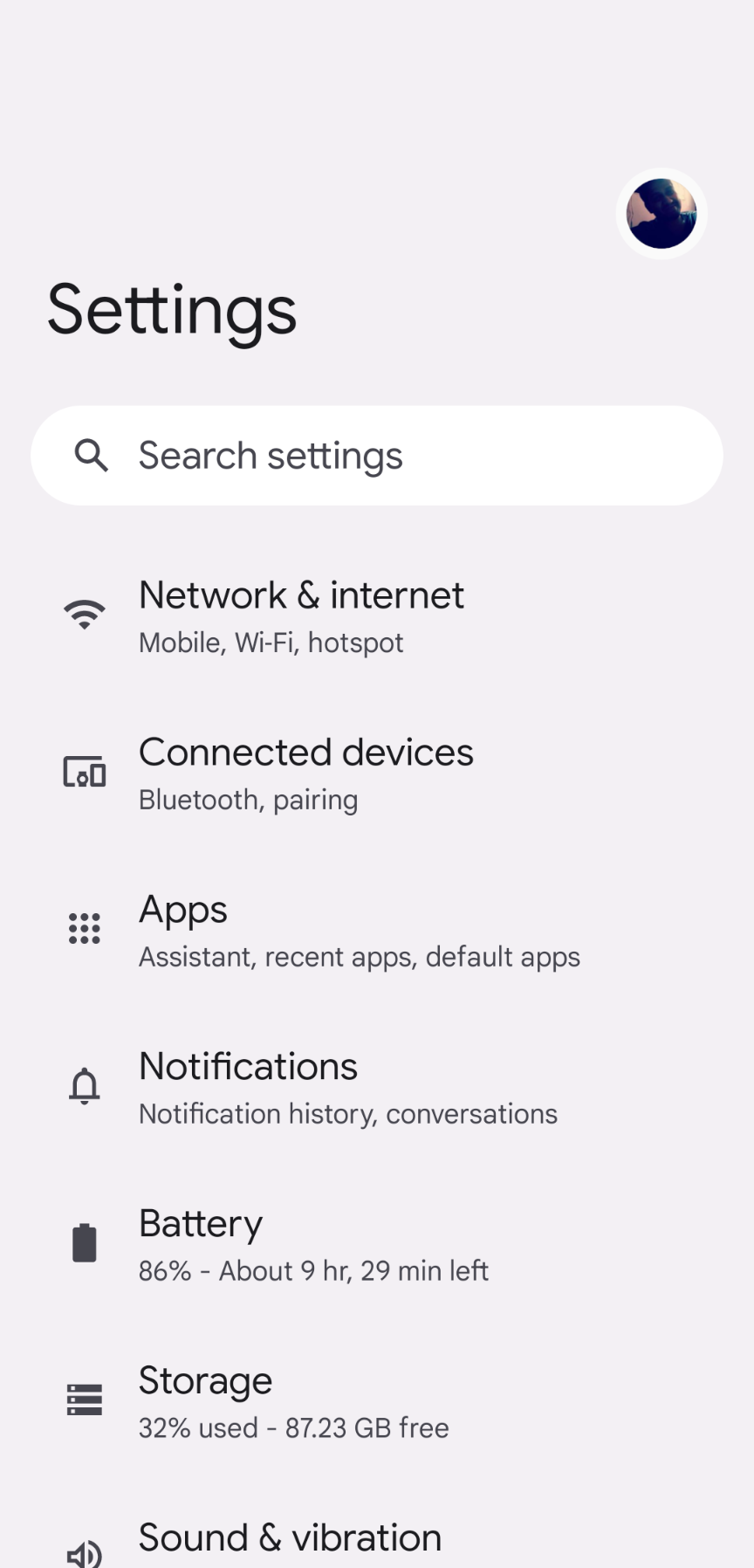The image displays a detailed view of the settings page on a smartphone. In the upper right corner, there is a circular profile picture with an image that is difficult to discern, possibly due to dark lighting, potentially of a person. Moving down, on the left side, the header prominently displays the word "Settings" in large black text.

Directly beneath the header, there's a search bar that includes a magnifying glass icon and the placeholder text "Search settings." Following the search bar, the layout continues with several categorized options:

1. **Network & Internet**: Icon of a wireless signal with text describing options such as "Mobile, Wi-Fi, Hotspot."
2. **Connected Devices**: Depicted with an icon showing several devices together accompanied by text including "Bluetooth, Pairing."
3. **Apps**: Represented by an icon of nine dots arranged in three rows and columns. The text elaborates options like "Apps, Assistant, Recent apps, Default apps."
4. **Notifications**: Featuring an icon of a bell, this section covers "Notification history, Conversations."
5. **Battery**: Illustrated by a battery icon displaying "86%" and "About 9 hours 29 minutes left."
6. **Storage**: Illustrated with three horizontal lines, it reads "32% used, 87.23 GB free."
7. **Sound & Vibration**: Depicted with an icon of a microphone with sound waves coming from it.

The background of the screen is a light gray color, and the overall shape of the device's screen is a tall rectangle.